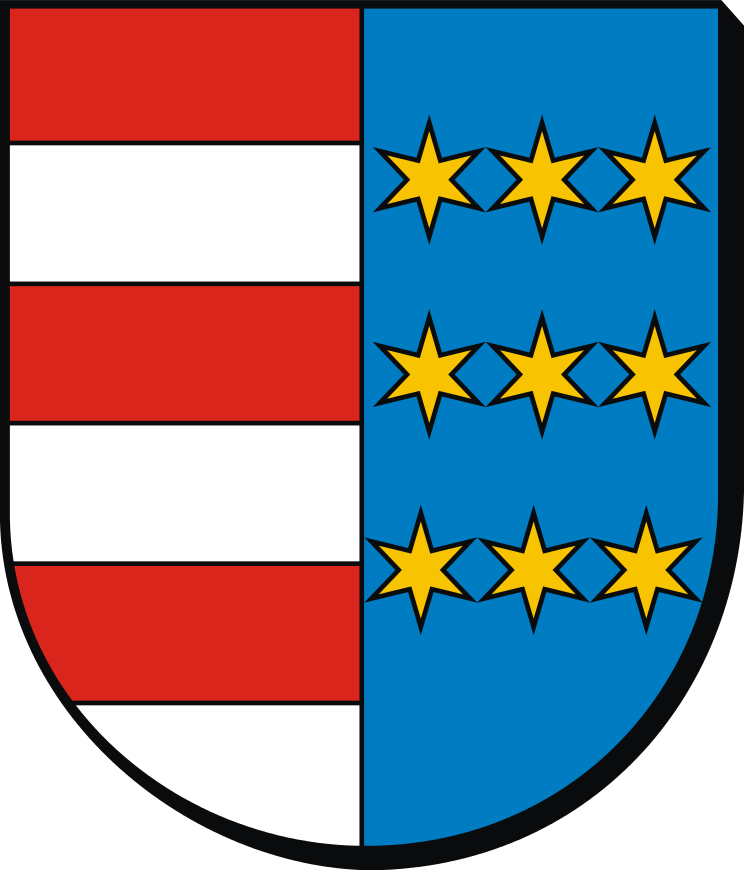The image portrays a cartoon-like drawing of a shield, resembling an upside-down tombstone or U-shape with a flat top. The shield is split vertically into two distinct halves. The left half features horizontal red and white stripes, each outlined in black, evoking the spirit of the American flag. The right half showcases a light blue background adorned with three rows of yellow, six-pointed stars, three stars in each row, all also outlined in black. A thin black line divides the two halves, and the entire shield is surrounded by a thick black border, lending it a three-dimensional appearance. This illustration, possibly set against a white background, combines elements reminiscent of heraldic crests and national symbols, blending them into a unique emblem.